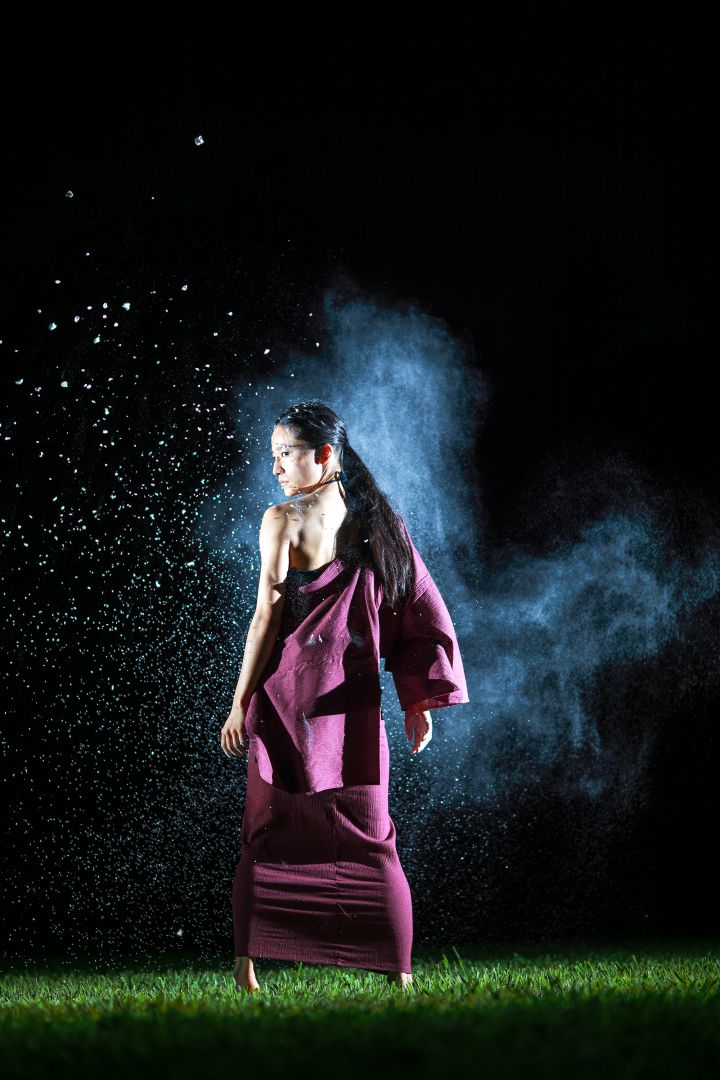In this striking full-color photograph taken outdoors at night, an Asian woman stands poised in a grassy field. The image, which is vertically rectangular and roughly twice as tall as it is wide, lacks a border and is enveloped in the deep blackness of the night sky. The green grass at the bottom forms a vivid contrast against the dark backdrop. The woman, positioned centrally, has her back to the camera but gazes over her left shoulder, revealing the left side of her face. Her long black hair is worn in a ponytail, cascading down to the middle of her back. She is adorned in a unique, dark purple dress that drapes to her ankles; the dress is distinctive for its asymmetrical design, featuring a full-length sleeve on the right while leaving her left shoulder and arm bare. A black garment peeks from under the robe on her left side. The scene is enhanced by a surreal ambiance of steam rising predominantly to her right, while on her left side, delicate droplets of water glisten, appearing like sparkles against the night.